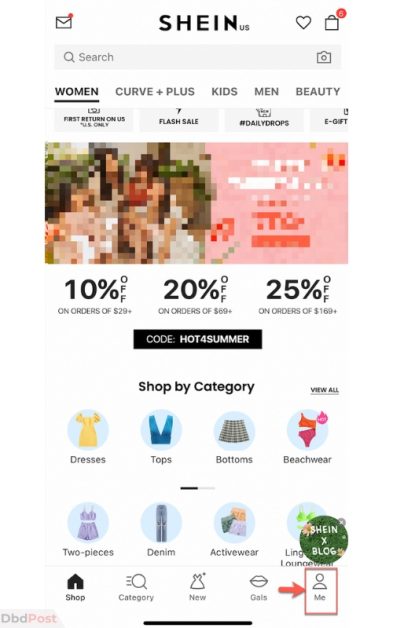This is an image showcasing the Shein website homepage. The layout is typical of an online shopping platform. Prominently positioned at the top-center is the Shein logo. Flanking it to the left is a message icon, and to the right are a heart icon and a share symbol. Directly below this header section is a search bar, which includes a camera icon on its right side for users to upload images.

Beneath the search bar, the navigation menu lists various categories such as Women, Curve + Plus, Kids, Men, and Beauty. Subcategories like Flash Sale, Daily Drops, and E-Gifts are situated below the primary categories for quick access.

What immediately draws attention is a large, prominently positioned image box within the upper middle section of the screen that appears completely blurred out. Typically, this could indicate restricted content, although the exact reason here is not specified.

Below this blurred-out section, several promotional deal banners are displayed, offering discounts ranging from 10% to 25% off. A promo code "HOTFORSUMMER" is provided, likely intended for new users to avail these discounts.

Further down the page, additional categories are segmented, including Dresses, Tops, Bottoms, and Beachwear. Each category is accompanied by a small emoji-type symbol representing its respective product type. The arrangement and visual cues guide the user seamlessly from top to bottom through the various offerings of the Shein website.